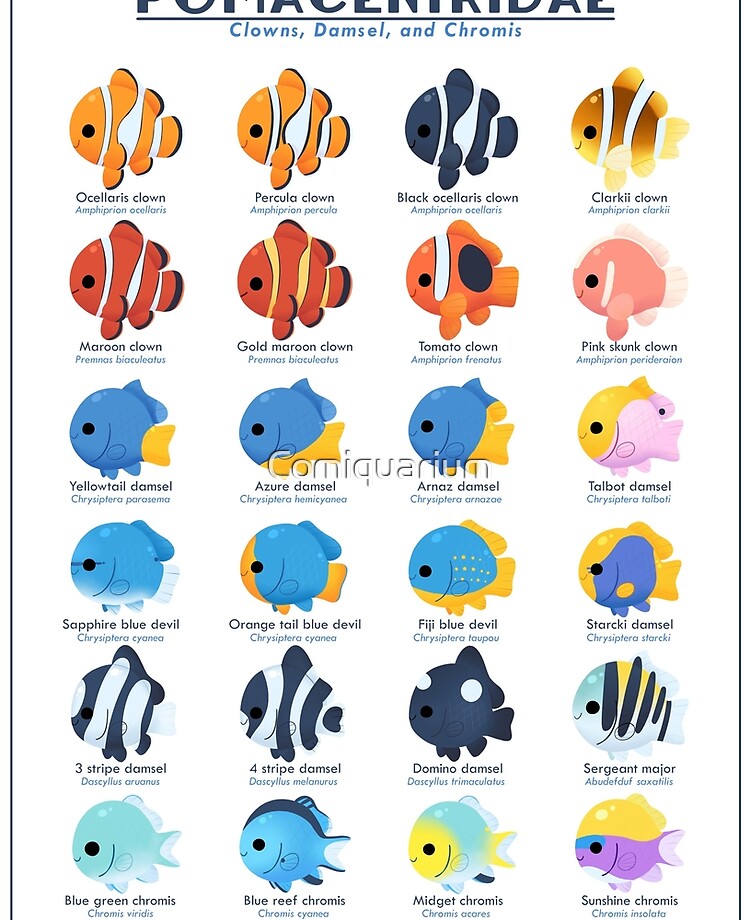This image is a detailed chart of various species of fish, organized in a grid of four columns across and six rows down. The chart highlights different types of clownfish in the first two rows, including species such as ocellaris clown, percula clown, black ocellaris clown, clarki clown, and pink skunk clown, which are predominantly orange with distinct patterns. The middle section features damselfish, which are typically blue. Species include the striped damsel, four-striped damsel, domino damsel, sergeant major, and starkey damsel. The final rows display a mix of damselfish and chromis species, with chromis fish like the blue reef and blue-green chromis mostly colored in blue hues. Each fish is illustrated with a cartoony style, showing their unique coloration and body part arrangement. Below each image, the fish's common name is in bold black text, and the Latin species name is in smaller italicized blue text. The chart is copyrighted by "Calm Aquarium," mentioned in the center, and the overall layout makes for a colorful and informative guide to these aquatic creatures.